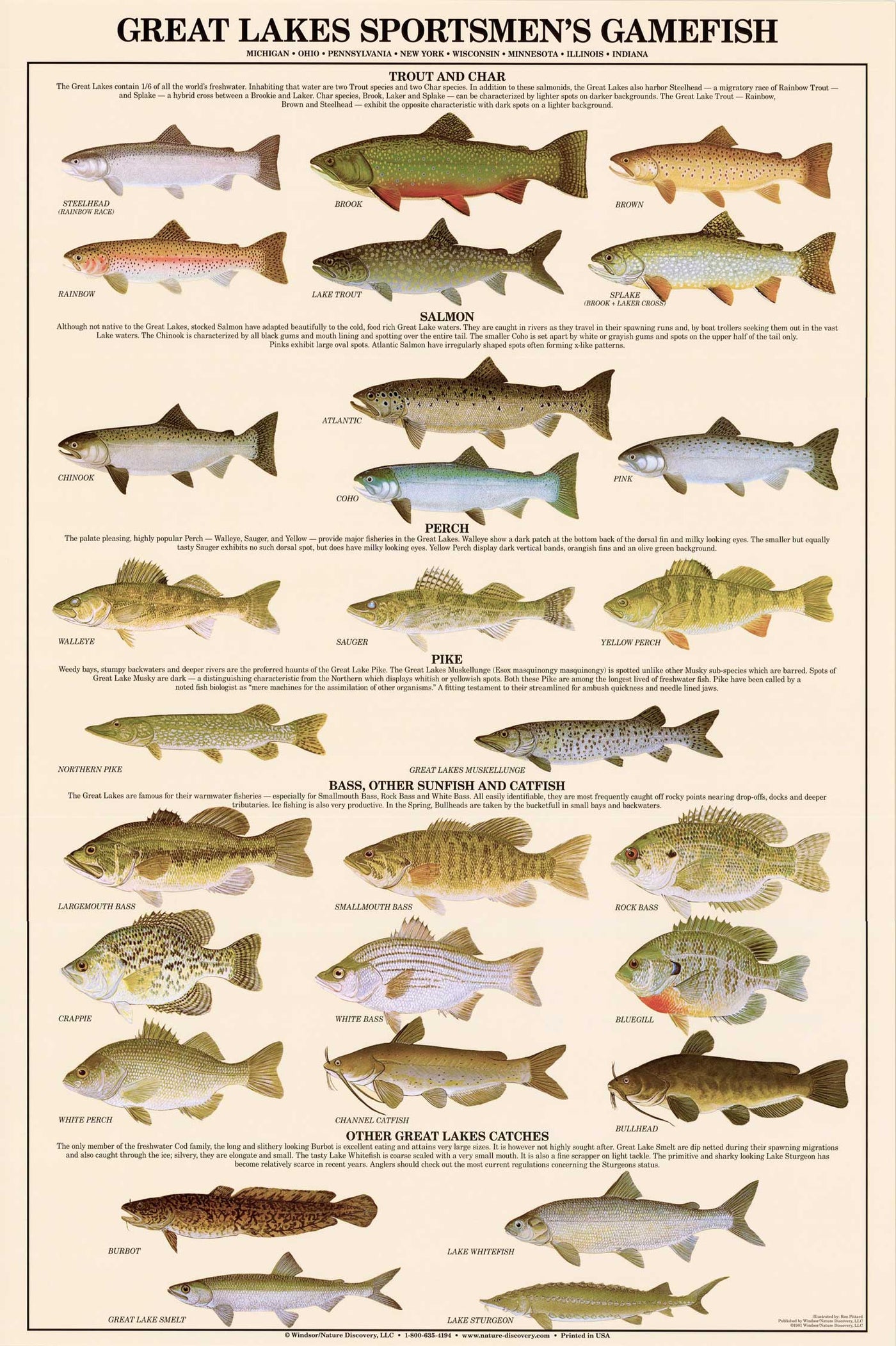This poster, titled "Great Lakes Sportsman's Game Fish," is an informative breakdown of various fish species found in the Great Lakes, elegantly illustrated and organized into distinct categories. The background of the poster is a beige hue, and its detailed illustrations give a vivid depiction of each fish. The title is prominently displayed in black text, and smaller, hard-to-read text offers additional information.

The poster is divided into several categories: "Trout and Char" highlighting six species; "Salmon" detailing four types of salmon; "Perch" with three different fish; and "Pike" featuring two fish. The category "Bass, Other Sunfish, and Catfish" showcases nine species, while "Other Great Lakes Catches" includes four distinct fish. Each fish is uniformly sized and oriented leftwards, with the species name and brief descriptions provided nearby. The overall design provides a comprehensive guide to the diverse game fish in the Great Lakes, making it both educational and visually appealing.